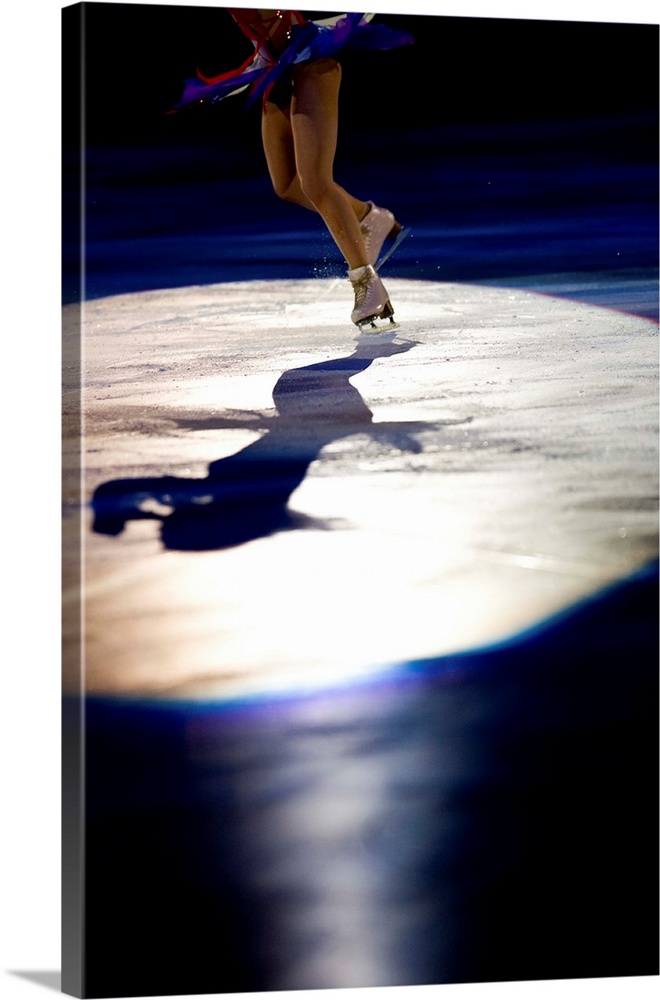The image captures a dramatic moment of an ice skating performance, portrayed on a rectangular monolith display. Bathed in the spotlight at an otherwise dark rink, a young female skater is the focal point. The light reveals her white ice skates with silver blades, her tan tights, and a vibrant tutu-style skirt adorned with red, white, and blue sequins. Her arms and torso are out of the frame, but her entire shadow stretches across the ice beneath her, hinting at the elegance of her movements. This dynamic scene, possibly set during a competition or public exhibition, appears to have been skillfully transferred onto a poster, which wraps around the monolith – likely made of wood, metal, or plastic. The depiction stirs a sense of motion and artistry, perfect for a decorative piece in a home.